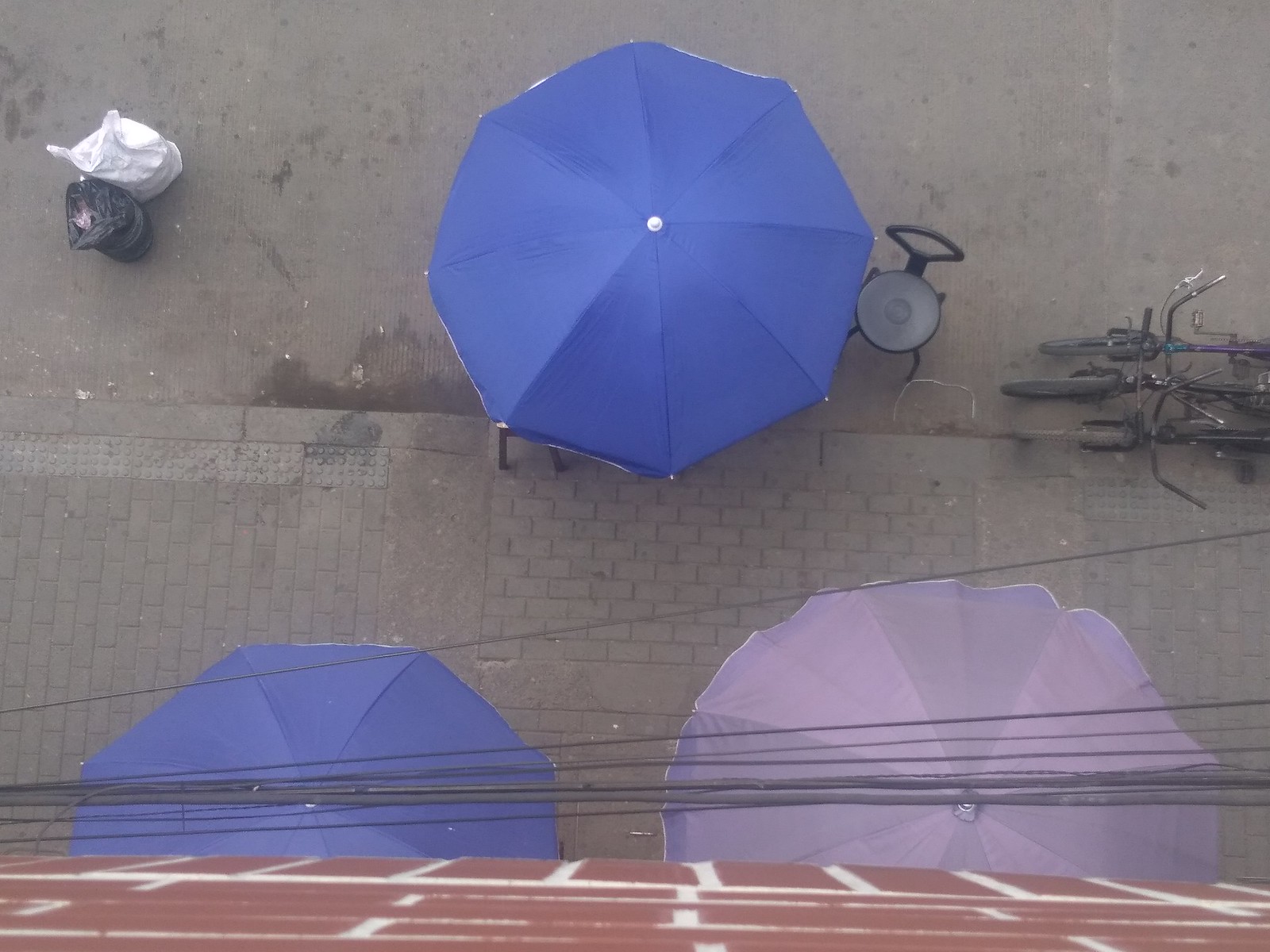This outdoor daytime photograph, taken from a second-story window on an overcast day, provides an overhead view of a street scene below. The lower part of the image shows a red brick wall belonging to the building from which the photo is taken. Directly below, a sidewalk bisects the image horizontally, giving way to a gray, slightly dirty paved street above it. Three large table umbrellas dominate the scene: a dark blue one partially visible on the left, a prominently placed purple one towards the center, and a fully visible green umbrella in the upper center. The green umbrella is accompanied by a green chair to its right. Overhead, horizontal communication and cable lines stretch across the view, represented as thin black lines. In the upper left corner, two bags of trash, one black and one white, are seen, and in the upper right, three tightly parked bicycles stand upright, suggesting a bike stand. These elements contribute to the impression of an open-air cafe or restaurant setting, despite no visible text or printing in the image.